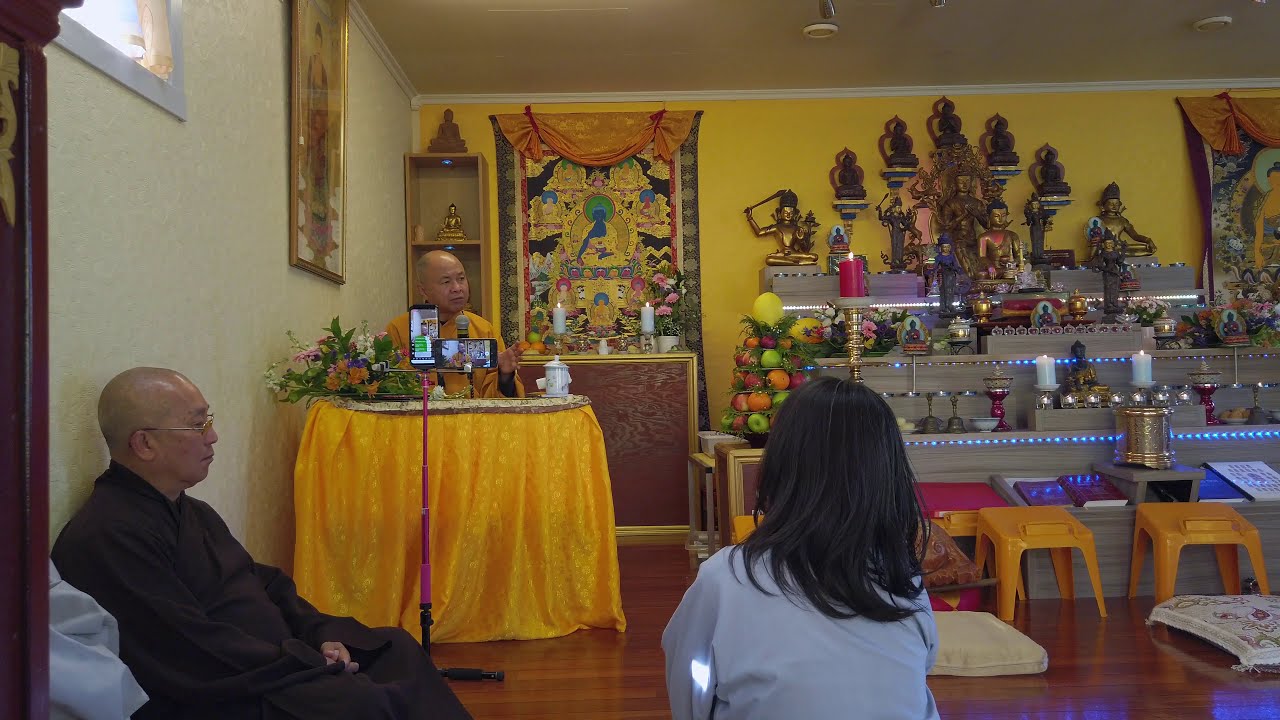The image depicts a serene indoor scene set in what appears to be a Buddhist temple, featuring three Asian individuals. The room has a horizontally aligned rectangular layout with a white wall on the left and a yellow wall in the background, adorned with ornate shelving. These shelves are gray in color and display an array of golden Buddhist monk statues, candles, and some fruit, with blue LED light strips accentuating the tiers.

On the left side of the image, a man with a bald head and wire-rimmed glasses wears a loose-fitting black robe. He sits with his back leaning against the white wall, gazing slightly forward. In the center of the image stands another bald man dressed in a yellow robe, seated behind a table draped with a bright yellow cloth that reaches to the floor. This table also holds a floral arrangement and has two phones set up, presumably for recording. There is a microphone positioned in front of him, and he appears to be looking slightly to the right as if addressing an audience or answering questions.

Toward the right of the image, a woman with long, straight black hair, wearing a gray long-sleeve top, is seen from behind, capturing only the upper part of her back. In the lower right-hand corner, a few plastic yellow stools are visible, set against a shiny wooden floor that adds a warm ambiance to the room. The overall scene is calm and contemplative, befitting a spiritual or meditative setting.